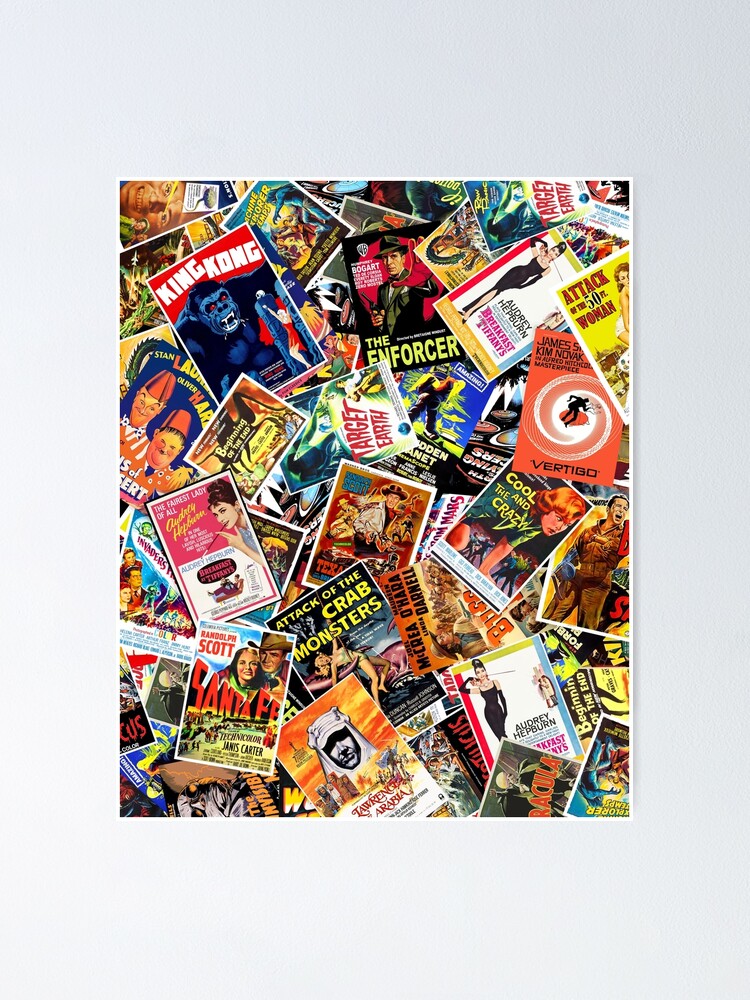The image features a rectangular collage pinned against a completely white wall, displaying a vivid array of vintage movie posters and magazine advertisements. The collage, bordered with a white edge, appears densely packed without any visible gaps between the items. Notable movie titles like *King Kong*, *Vertigo*, *Attack of the Crab Monsters*, *Santa Fe*, *Dracula*, *The Enforcer*, and *Breakfast at Tiffany's* appear prominently amidst a colorful amalgamation of 1950s and 60s advertisements, including some promoting cigarettes to women. The posters are piled from the bottom to the top, combining to create a nostalgic mosaic of classic cinema and mid-century print media. The collage's vibrant hues of red, pink, yellow, and orange contribute to the overall vintage aesthetic, reminiscent of a bygone era in film and advertising history.